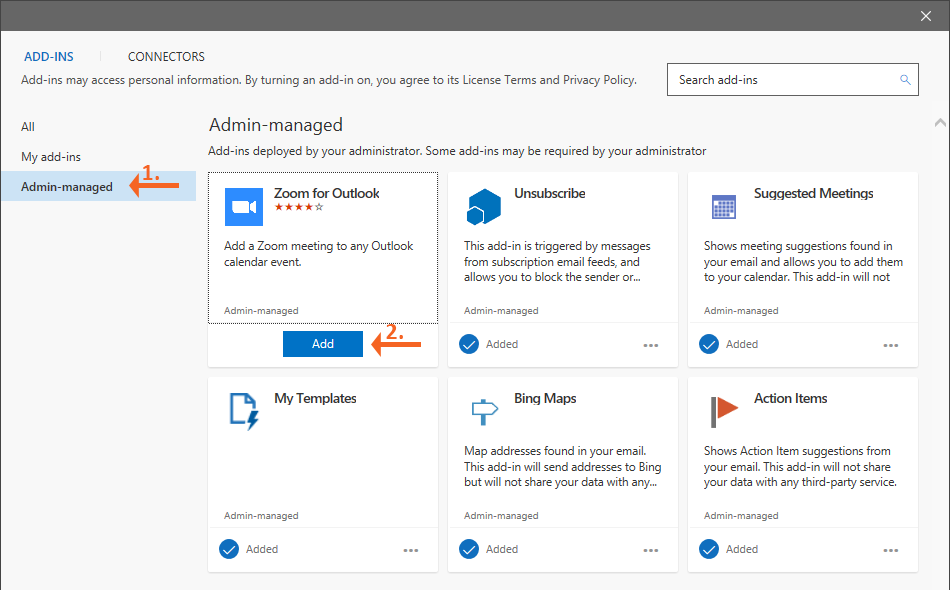The image displays a section of a Microsoft app store, specifically focusing on add-ins and connectors. At the top of the page, there is a notification indicating that add-ins may access personal information and that by installing an add-in, you agree to its license terms and privacy policy. A search bar is situated to the right of this notification. 

On the left side, there's an option to select "All My Add-ins" or "Admin Managed Add-ins." The "Admin Managed Add-ins" option is selected, as indicated by a number one and a red arrow pointing to it, denoting it as the first step. 

The central portion of the screen is organized in a grid layout, displaying various admin-managed add-ins. Visible add-ins include "Zoom for Outlook," "Unsubscribe," "Suggested Meetings," "My Templates," "Bing Maps," and "Action Items." Except for "Zoom for Outlook," all these add-ins are already installed, which is highlighted by a red arrow pointing to the "Add" button below the "Zoom for Outlook" add-in, labeled as step two.

The description next to the "Zoom for Outlook" add-in reads: "Add a Zoom meeting to any Outlook calendar event." The icon for this add-in is a blue square with a white camcorder symbol in the center.